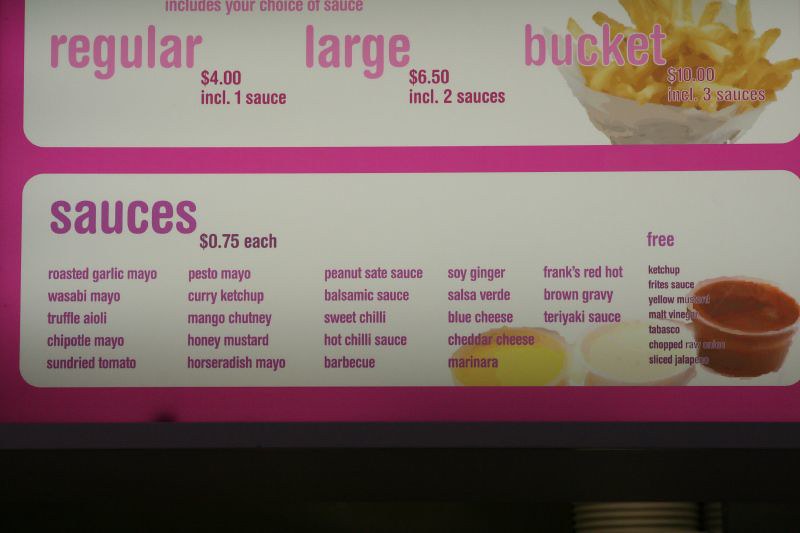### Detailed Caption

A vibrant, color photograph captures a well-lit menu sign on the wall of a fast food restaurant. The menu features a white background with a striking hot pink border that divides its sections and adds a lively touch to the overall design. On the right side of the sign, a colorful image of golden French fries nestled in a paper cone entices customers, though the top part of the image is slightly cropped out of the frame. 

Beneath this image, the menu offers a "Bucket" of fries priced at $10, which includes three sauces. Adjacent to the bucket option, on the left, are additional choices: a "Regular" serving for $4 with one sauce included, and a "Large" serving for $6.50 that comes with two sauces. 

The bottom section of the sign, written in various shades of pink and magenta, lists an array of available sauces priced at 75 cents each. These sauces include Roasted Garlic Mayo, Wasabi Mayo, Truffle Aioli, Chipotle Mayo, Sun-Dried Tomato Pesto Mayo, Curry Ketchup, Mango Chutney, Honey Mustard, Horseradish Mayo, Peanut Satay Sauce, Balsamic Sauce, Sweet Chili, Hot Chili Sauce, BBQ, Soy Ginger, Salsa Verde, Blue Cheese, Cheddar Cheese, Marinara, Frank’s Red Hot, Brown Gravy, and Teriyaki Sauce. Additionally, a selection of free sauces is provided, featuring Ketchup, Yellow Mustard, Malt Vinegar, Tabasco, and sliced Jalapeños, though some details in this section are difficult to read due to the small text size.

Adding to the visual appeal, an illustrated trio of translucent dipping cups showcases a variety of sauces, one resembling cheese, another a mayo-based dip, and the third appearing as classic ketchup. Beneath the menu sign, a darkened shelf holds a stack of plates, partially visible but shrouded in shadow, further contributing to the bustling and inviting atmosphere of the restaurant.